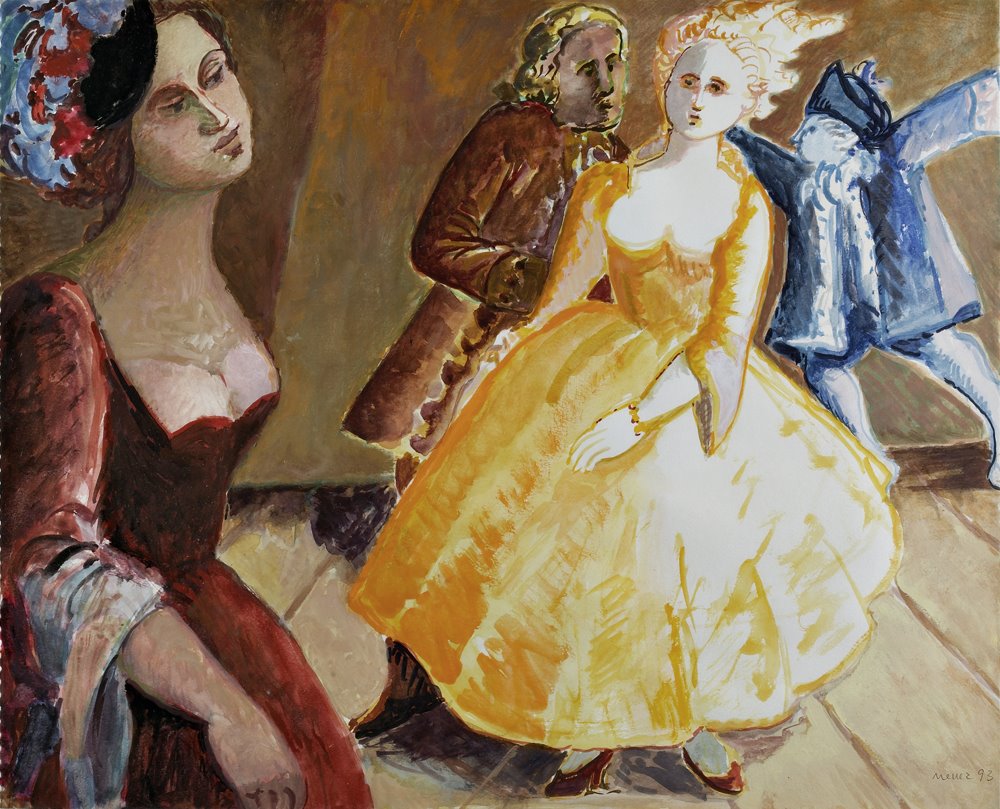This hand-painted piece exudes an abstract yet subtly realistic vibe, suggesting an 18th-century setting through the attire of its depicted figures. Dominating the foreground on the left, a woman with light skin and black hair adorned with red and blue feathers strikes a commanding presence in a striking red dress with open sleeves and a sweetheart neckline. Her right arm is positioned in front of her, and she gazes off to the right. Centrally, a blonde-haired woman with a round face stands out in a resplendent yellow ball gown with a sweetheart bodice. Her right arm is similarly positioned in front while her left is slightly obscured behind her. To her left, encroaching upon her personal space, is a man with a white wig and an old, formal red jacket reminiscent of a British officer from the Revolutionary War. In the right background, a small figure dressed entirely in blue—including a colonial-style tricorn hat and an intricate overcoat—adds a peculiar, almost ghostly touch to the scene. The painting, filling nearly the entire frame, sits atop a hardwood or tile floor, and its palette encompasses light and dark browns, blues, reds, yellows, and whites. The signature “Menez, '93” or “Muez, '93” inscribed in the bottom right corner further authenticates this intricate and detailed artwork, merging historical essence with abstract expression.